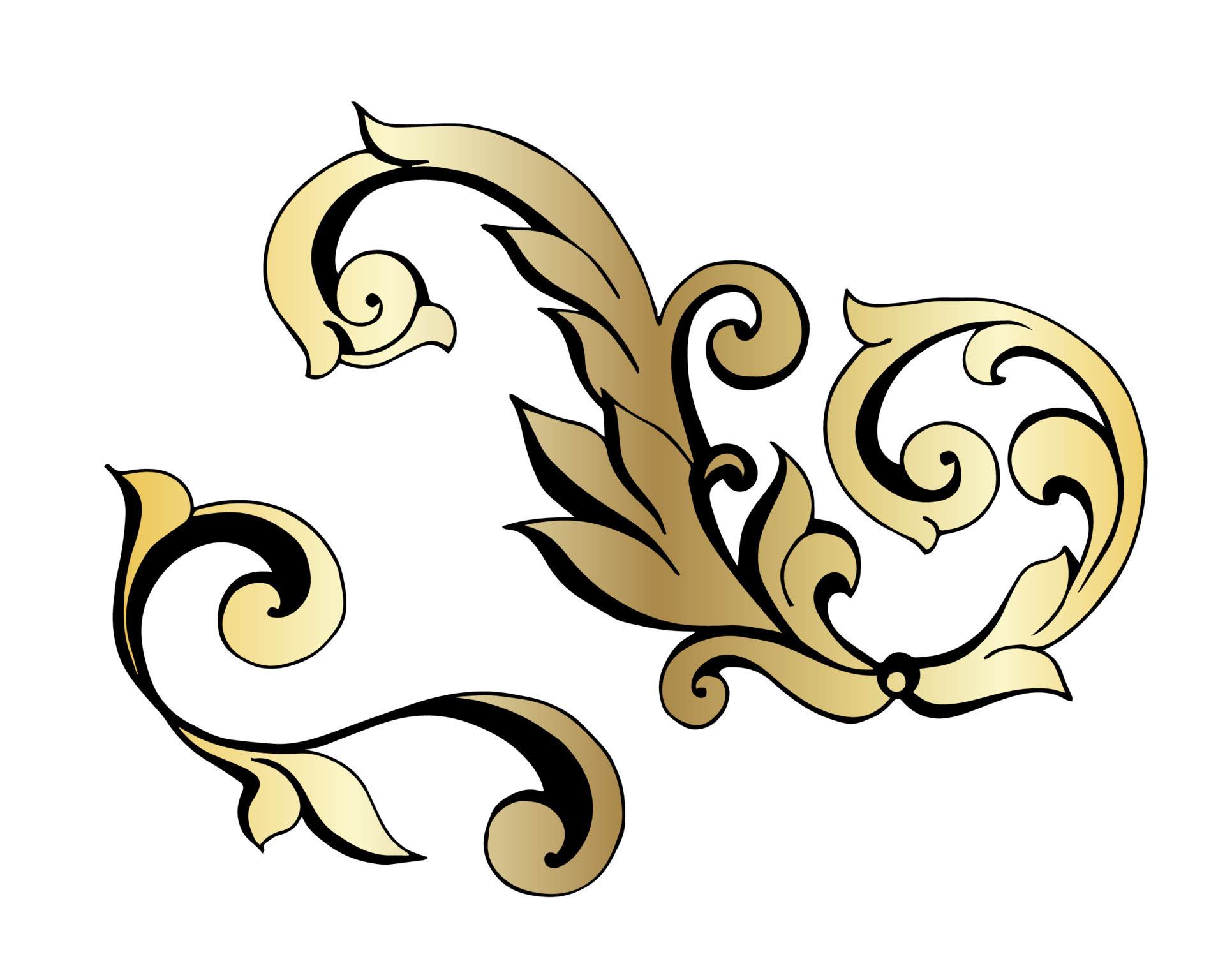This image features an intricate, hand-drawn or computer-animated design set against a plain white background. The composition includes two ornate, S-shaped patterns, one significantly larger and more elaborate in the top right corner and a smaller counterpart in the bottom left. Both designs incorporate fluid, swirling lines reminiscent of leaves, ribbons, and curlicues, with detailed flourishes similar to a more elaborate fleur-de-lis. The patterns are outlined in bold black and filled with gradient shades of gold, ranging from dark to light, giving them a rich, dimensional appearance. The overall style suggests a decorative motif suitable for inclusion in a larger art piece or as an embellishment on a tile.